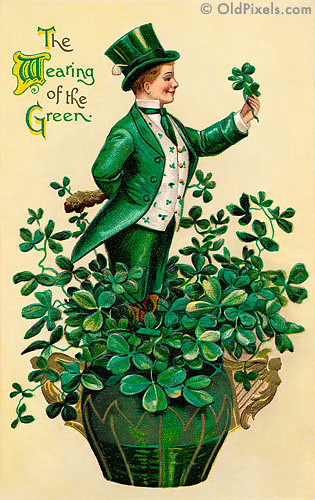This vintage illustration titled "The Wearing of the Green," from oldpixels.com, features a whimsical leprechaun figure standing within a green vase adorned with gold, harp-shaped handles, and outlined in a jagged golden shape against a beige background. Emerging from the vase are lush green clovers. The leprechaun is dressed in a vibrant outfit, complete with green pants and an open green jacket over a white shirt printed with green leaves. He sports a matching green top hat accentuated with a white pipe in the band and a green necktie. His rosy cheeks, pink lips, and short orange hair give him a cheerful appearance as he smiles warmly. In his left hand, he holds a single clover, while his right hand, tucked behind his back, clutches a brown rabbit’s foot. The upper left corner of the image displays the phrase "The Wearing of the Green" in old-fashioned text with alternating green and black letters. A gray watermark reading "©oldpixels.com" is positioned in the top right corner, adding a touch of authenticity to this nostalgic and joyful depiction.